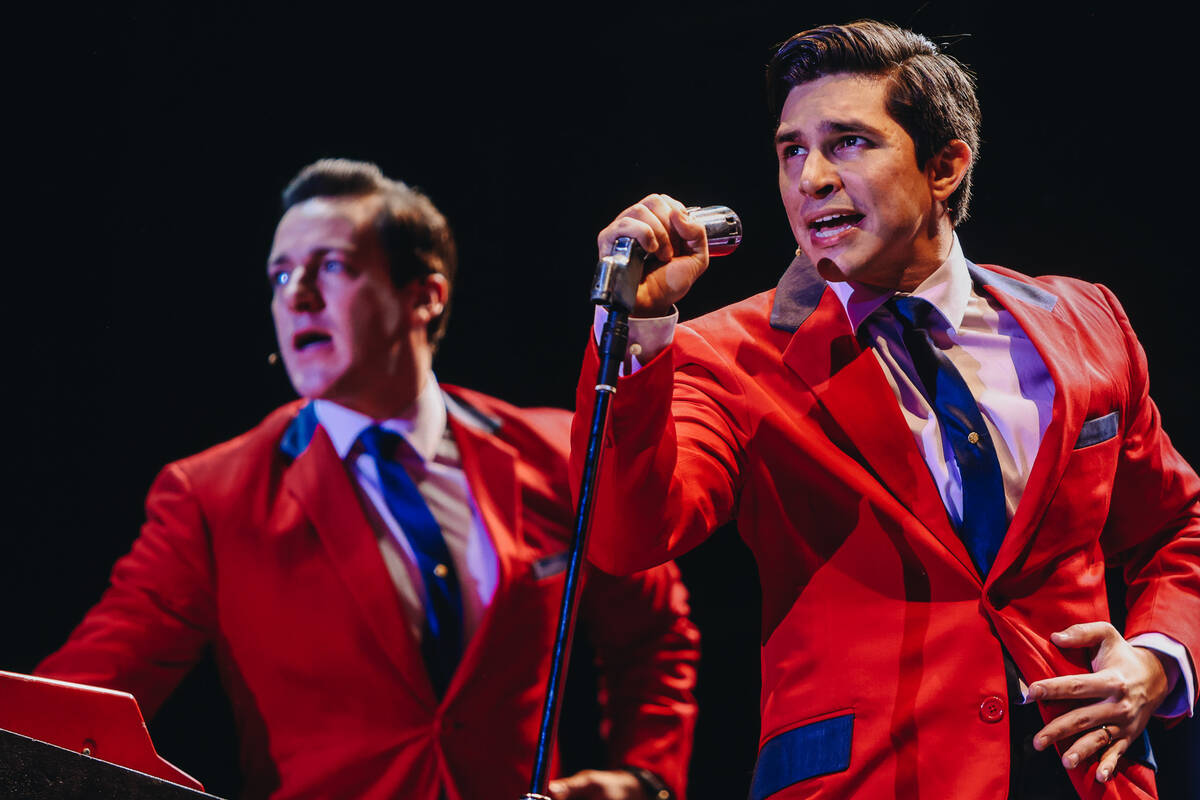In the image, two young men, both wearing bright red suit jackets accented with blue highlights on the collar and pocket areas, are performing against a completely black background. They each sport white dress shirts and blue ties, the latter adorned with small gold tie clips. One man, positioned slightly in front, is holding a microphone affixed to a blue stand that matches the blue details in their attire. The other man appears to be using a head-mounted microphone, though it's not immediately visible. Both seem to be singing, with the front man intently looking towards the upper left. A music stand, possibly holding lyrics or sheet music, can be spotted in front of them. The combination of their matching outfits and the setup suggests a coordinated performance, potentially from a concert or movie scene.